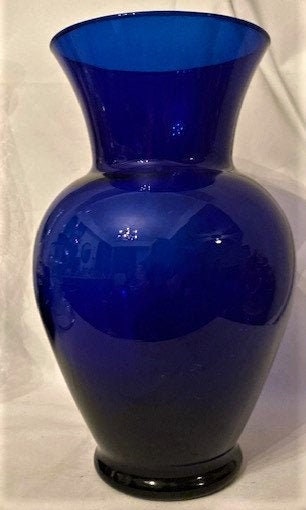This photograph showcases a royal blue glass vase set against an off-white fabric background that is wrinkled in the upper right-hand corner. The background casts blue-gray shadows, adding depth to the scene. The vase itself is semi-translucent with a thick, rounded base leading up to a wider, bulbous bottom that narrows into a slender neck before flaring out slightly at the top. There are no flowers inside the vase, allowing its striking blue color and elegant form to take center stage. The vase reflects light from an overhead chandelier-style fixture and contours of the surrounding room, suggestive of a living space, though specifics of the room's furnishings remain indistinct. Light spots and reflections trace the vase's contours, creating an interplay of light and shadow that enhances the visual complexity of the scene.